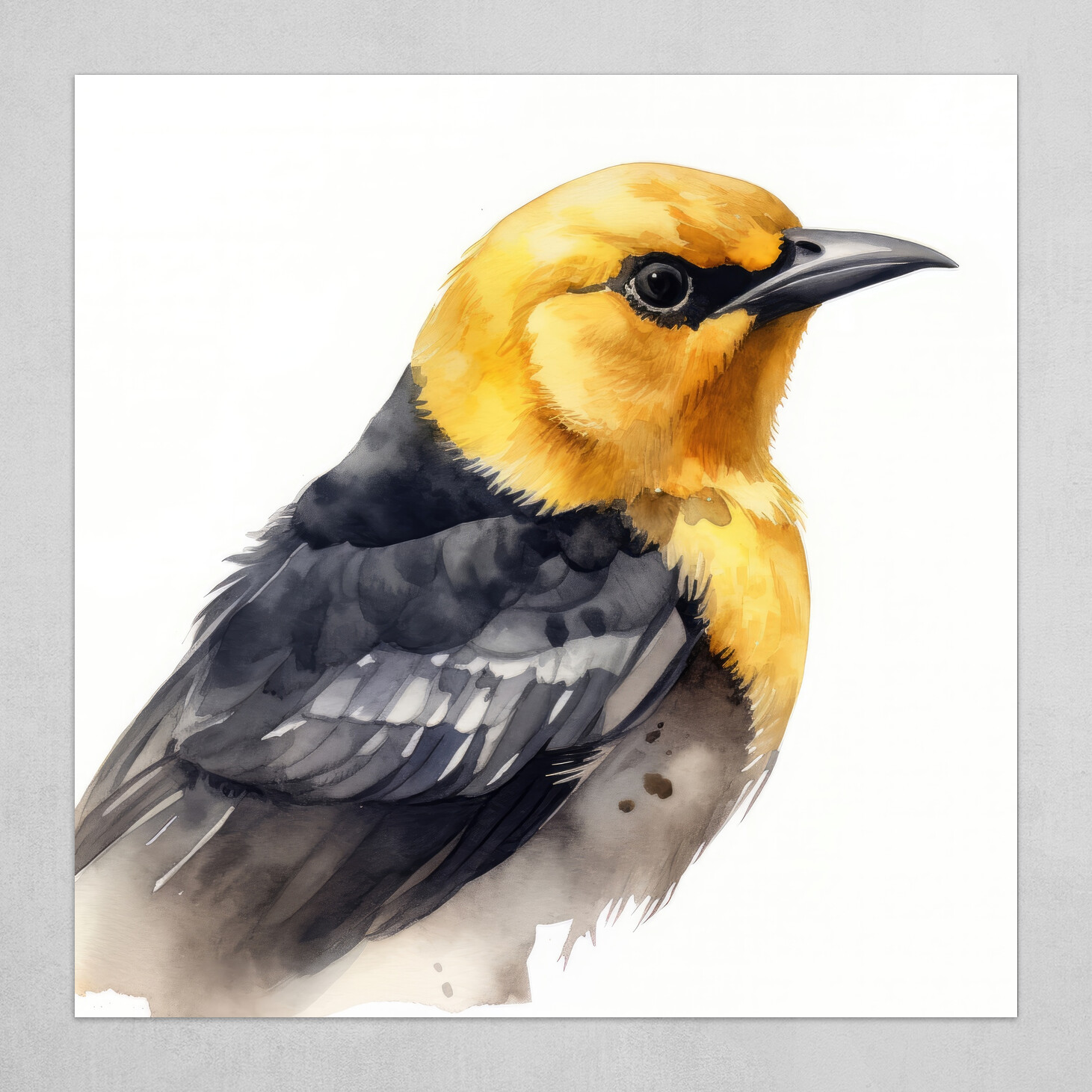This is a watercolor painting of a bird depicted in a semi-realistic style, showcasing its head and upper body with a vivid attention to detail. The bird, standing and facing towards the right, has a strikingly vibrant yellow-orange head crowned by a sharp, focused black eye. Surrounding the eye, the feathers gradate from the bright yellow-orange to a soft off-white before deepening to black around the beak and the back of the head. Its beak is sharp, black, and slightly curved, characteristic of many bird species. The bird's neck and upper body are adorned with intricately rendered gray and black feathers, showcasing an array of individual feather details that highlight the texture and layering of its plumage. The wings exhibit a subtle transition from grayish tones to white, complementing the lighter coloration of its belly. The painting's composition does not reveal the bird's legs or feet and is cut off just before the tail, offering a focused view of its torso. The artwork is set within a gray border, approximately an inch thick, against a completely white background, further emphasizing the bird's vibrant and lifelike appearance.